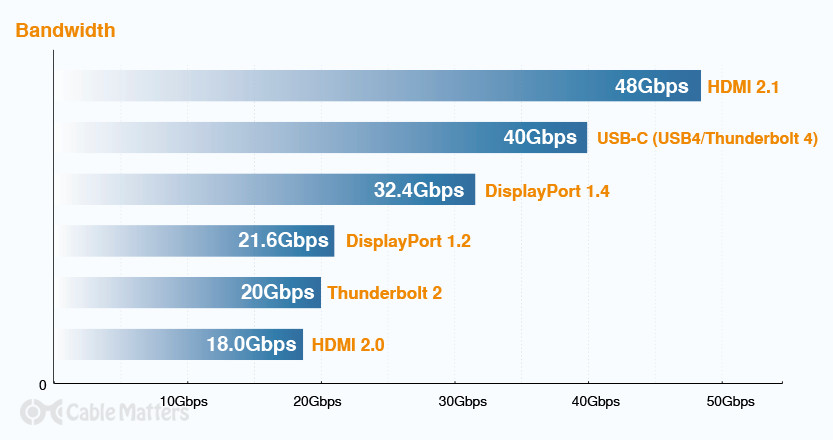This digital infographic features a detailed bar chart illustrating the bandwidth capacities of various connector types. The image includes a thin black border on the left side and bottom, along with a watermark in the lower left-hand corner marked by a glasses-like symbol and the text "Cable Matters." 

In the upper left corner, the chart is labeled "Bandwidth." The vertical axis measures bandwidth, scaled from 10 to 50 gigabits per second (Gbps) in increments, while the horizontal bars, shaded in gradient blue from gray-white on the left to dark blue on the right, represent the data for different connector types. The infographic shows:

- HDMI 2.1 with a bandwidth of 48 Gbps at the top.
- USB-C, USB 4, Thunderbolt 4 with a bandwidth of 40 Gbps below it.
- DisplayPort 1.4 at 32.4 Gbps.
- DisplayPort 1.2 at 21.6 Gbps.
- Thunderbolt 2 at 20 Gbps.
- HDMI 2.0 at the bottom with 18 Gbps.

Each bar's length corresponds to its bandwidth, providing a visual comparison of the data transmission speeds for these connectors.